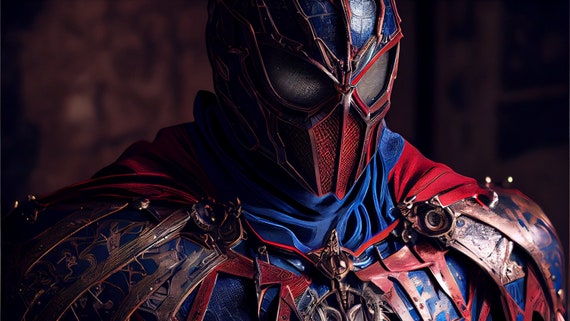This is a detailed color photograph featuring an individual dressed as a superhero. The person’s face is completely obscured by a helmet that combines blue and red hues and is distinguished by large, opaque eye areas. The costume includes blue accents around the collar and a dramatic red cape that cascades behind them. The front of their uniform is fortified with bronze-colored armor, prominently displaying a shield emblem at the center, though the bottom part of the emblem is not visible within the frame. The backdrop is dark and blurred, drawing focus to the vivid superhero costume. The landscape orientation of the image emphasizes the width over the height. The image is devoid of any text, animals, plants, flowers, trees, or motorized vehicles, ensuring all attention is on the superhero figure.